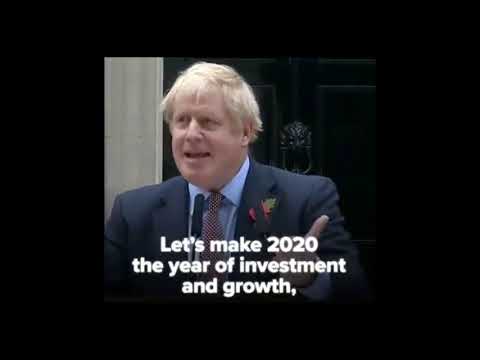The image primarily features British Prime Minister Boris Johnson, who is positioned directly in the center. He is characterized by his typical messy blonde hair and is dressed in a suit. The background shows the iconic location of 10 Downing Street. The image includes a text statement located at the bottom, which reads: "Let's make 2020 the year of investment and growth." This text is white and set against a black outline of a square. The right side of the image is largely occupied by a door, and there is a wall visible on the left. Surrounding the entire image is a border. The color palette of the image includes black, off-white, gray, light blue, maroon, green, orange, and yellow. The overall setting and style suggest that this image is designed for circulation on social media, possibly with a meme-like quality.